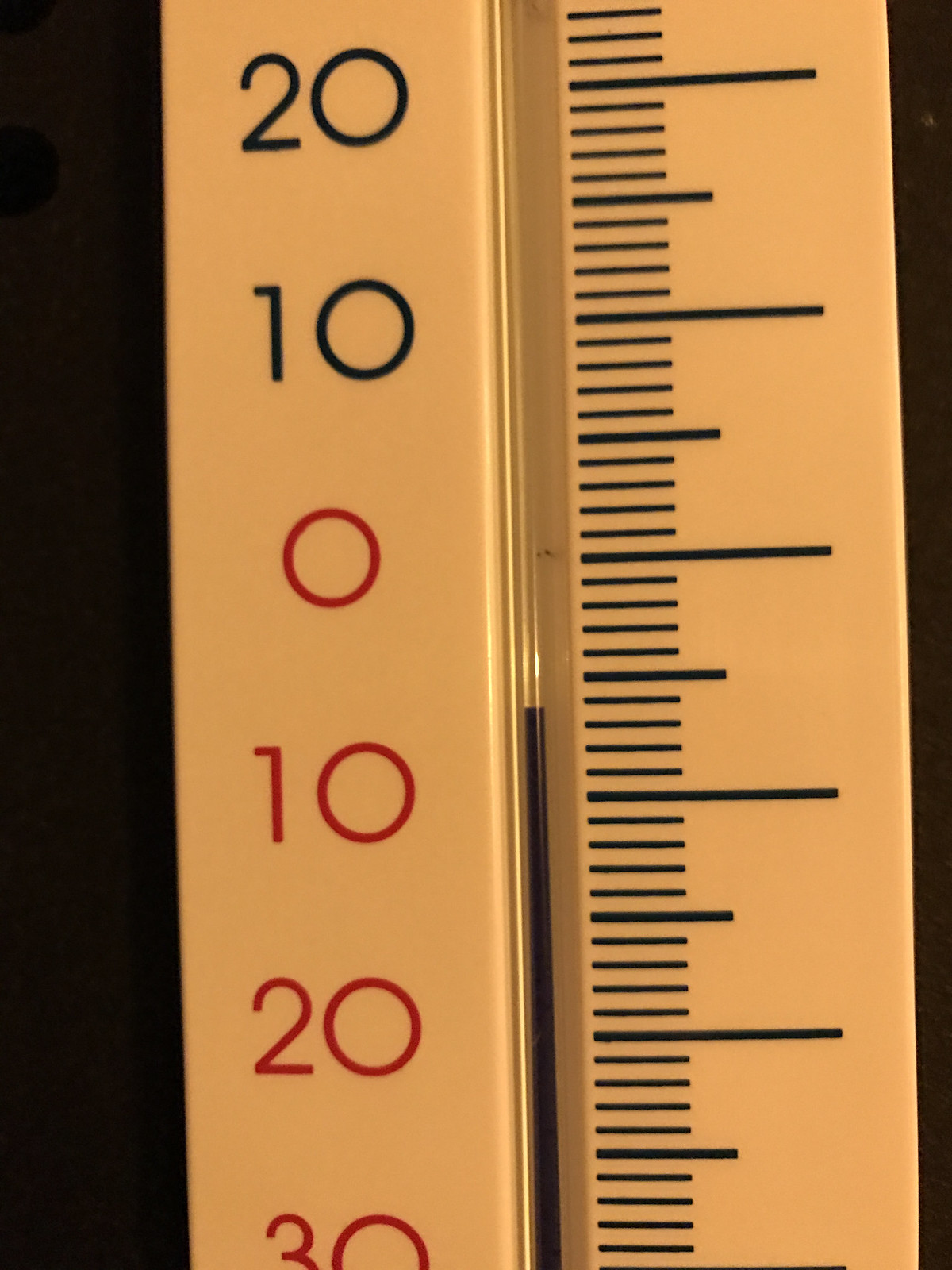The image is an extreme close-up view of a thermometer, so zoomed in that it captures only the segment from approximately the 23°C mark at the top to the -30°C mark at the bottom. The numbers on the thermometer are positioned on the left side, with the markings for 20, 10, and 0°C in black, while the markings for -10, -20, and -30°C are in red. The thermometer itself appears to be an orangish-beige color due to the extreme zoom, though it likely is white under normal lighting conditions. 

On the right-hand side, black tick marks indicate every 10-degree interval prominently, with semi-predominant marks at every 5-degree interval. The current temperature reading, indicated by the black mercury in the center, is approximately -6°C. The thermometer's close-up emphasizes the fine details and textures, and the unusual black mercury adds a unique twist to the traditional red color typically seen in thermometers.